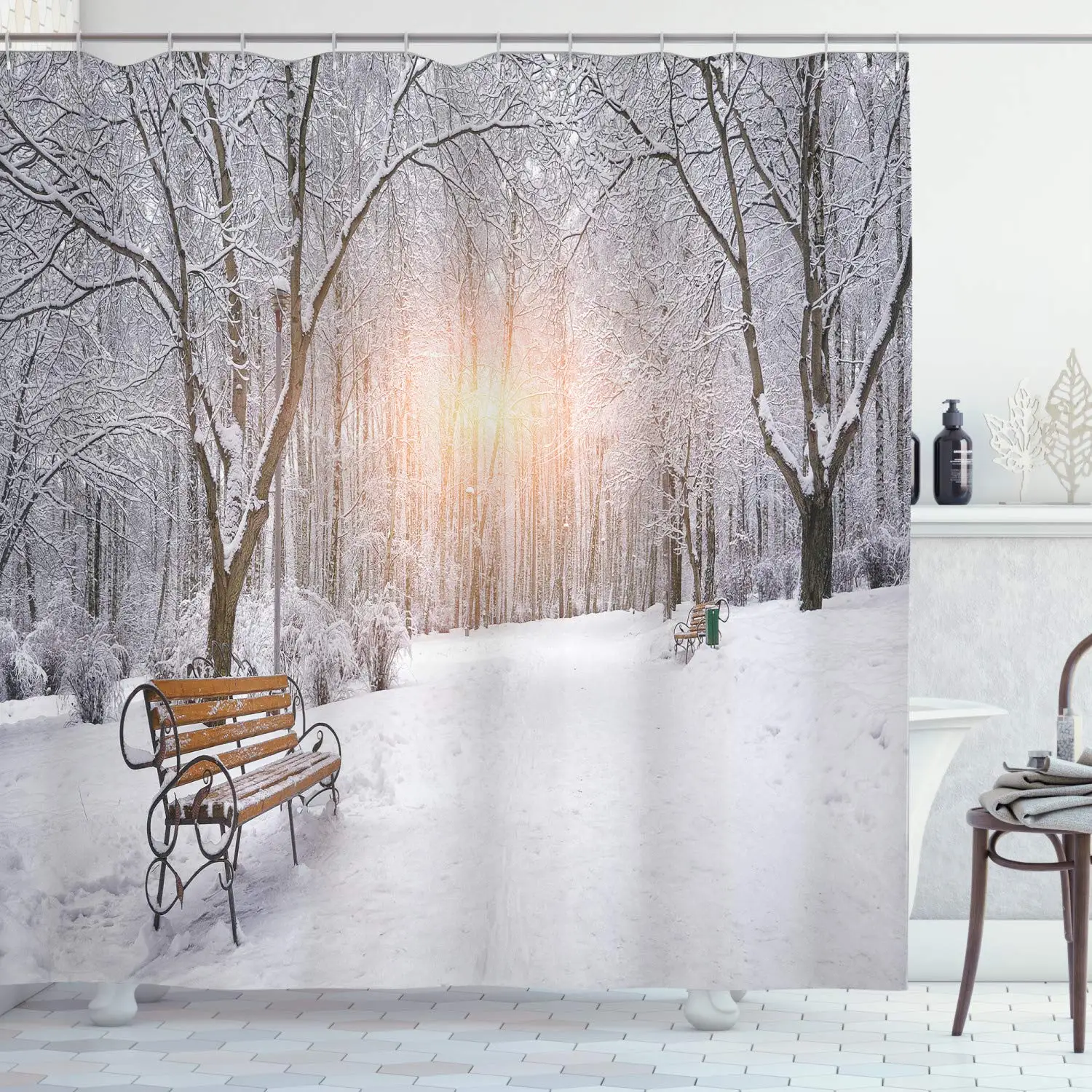The image is of a shower curtain hanging in a white-tiled bathroom. The shower curtain features a detailed winter scene with snow-covered ground and a slippery-looking walkway stretching out in front. On the left side, there's a wooden bench with intricate wrought iron, flanked by some smaller snow-laden plants. Further back on the right-hand side, another park bench sits down the path. Dominating the background are very tall trees, all blanketed in snow, with their branches reaching skyward. Between the tree trunks, the sun shines through, casting a reddish glow that contrasts with the cold, snowy surroundings. Inside the bathroom, there's a silver pole with silver hooks supporting the curtain, a shelf above holding some brown bottles, and a chair with towels placed on its seat peeking out from the right-hand corner.